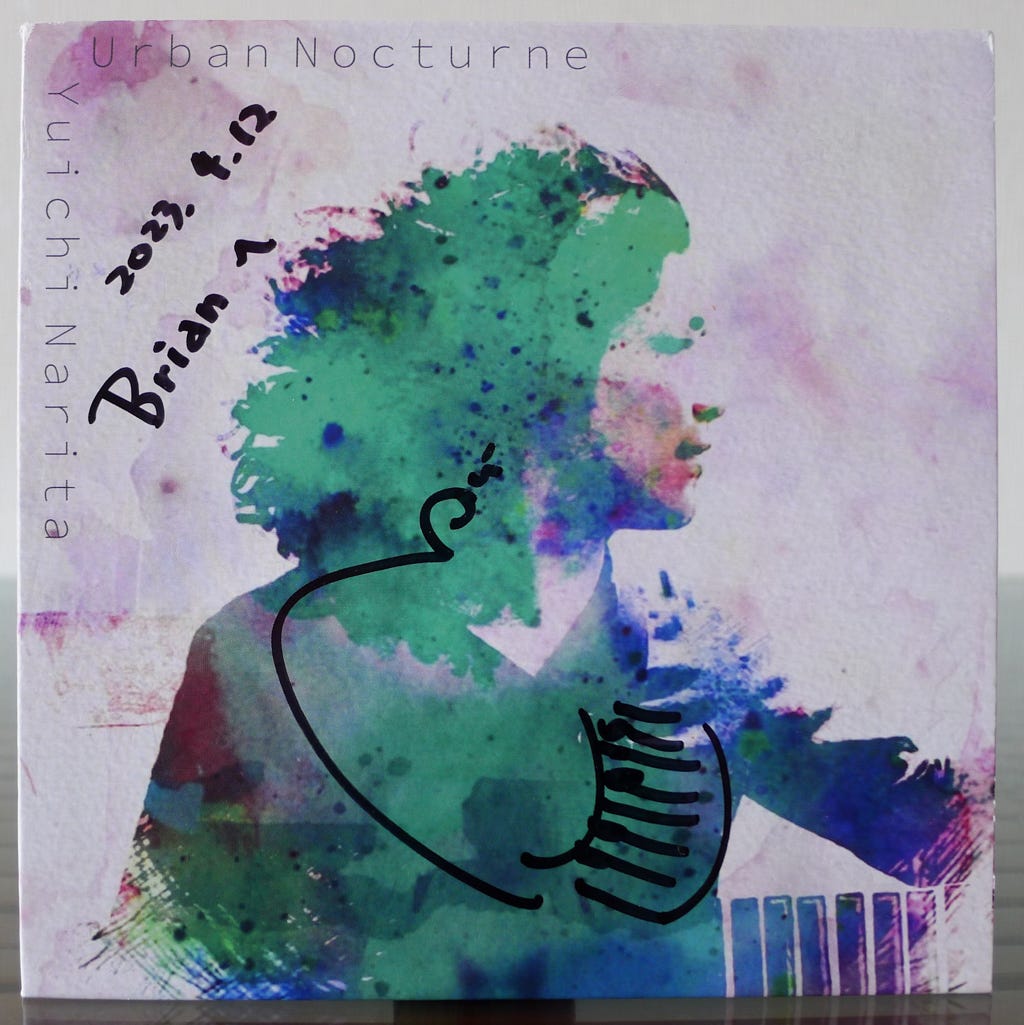The image showcases a close-up photograph of what appears to be an album cover for a vinyl record. At the top, in thin, light blue text, it reads "Urban Nocturne." Vertically aligned on the left side is the name "Yuichi Narita," written in the same font. Below this, handwritten in Sharpie, is the date "2023.4.12" alongside the name "Brian" and a squiggly mark. The vinyl features an artistic depiction of an individual gazing to the right, set against a tie-dye, sunset-inspired background with hues of pink, white, green, purple, blue, and black. The artwork blends splotchy paint and smooth strokes, along with some black lines that may represent a necklace. The person in the image, characterized by light facial features and flowing hair, appears androgynous and is wearing a shirt. The bottom right side of the cover includes a series of rectangles or blocks arranged horizontally.